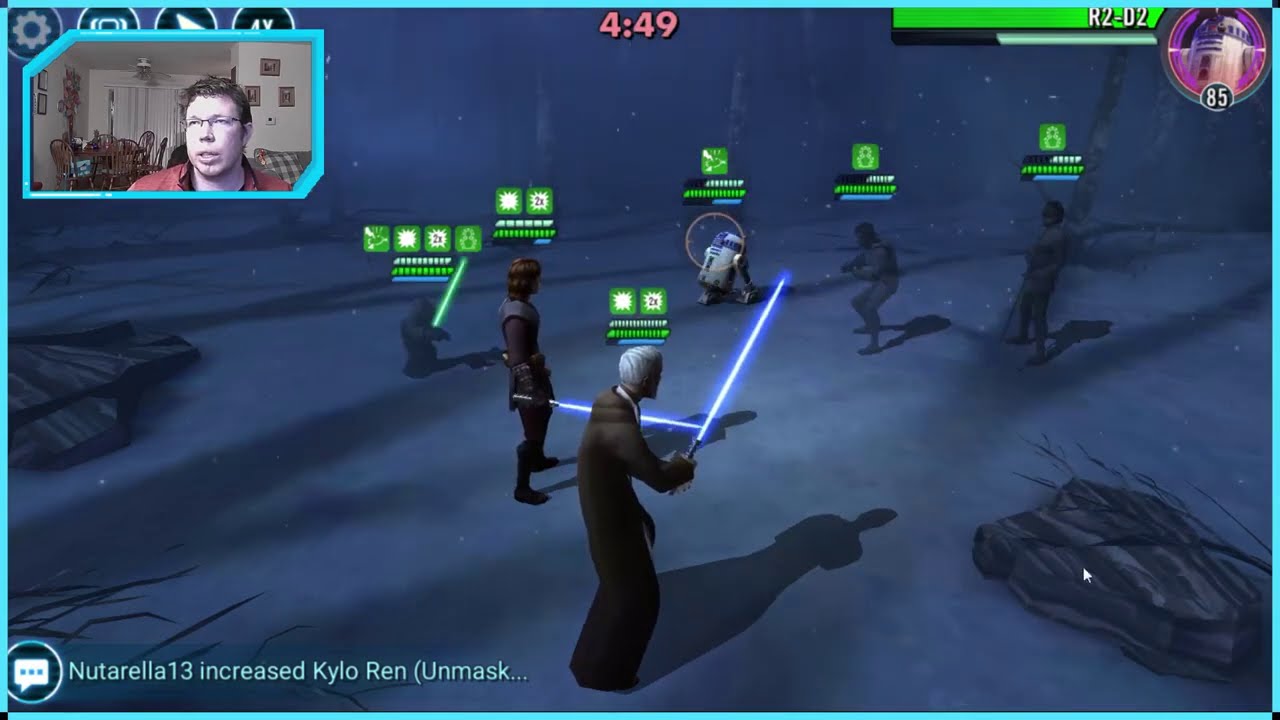The image is a detailed screenshot from a video game being streamed by a player who's visible in a blue-outlined inset in the upper left-hand corner. The player, a Caucasian male with short brown hair, glasses, and a red shirt, is situated in his living room, with a dining set visible behind him. The main portion of the screen features recognizable Star Wars characters in a snowy field, seemingly preparing for a battle.

On the right side of the screen, an older Obi-Wan Kenobi, with gray hair and a brown robe, wields a blue lightsaber. Next to him, Anakin Skywalker, dressed in dark clothing, also brandishes a blue lightsaber. Yoda, the tiny green Jedi, stands to their left holding a green lightsaber. They are facing off against R2-D2 and two other indistinct, transparent figures yet to be chosen by players.

In the upper center, the time is displayed as "4:49" in pink text. The upper right corner contains a health bar labeled "R2-D2" with a green stripe and the corresponding droid image, indicating the health is at 85. The lower left corner features a chat bubble with the text, "Nuterella 13 increased Kylo Ren unmask…". The overall setting is a futuristic, dark blue landscape, typical of a video game environment.